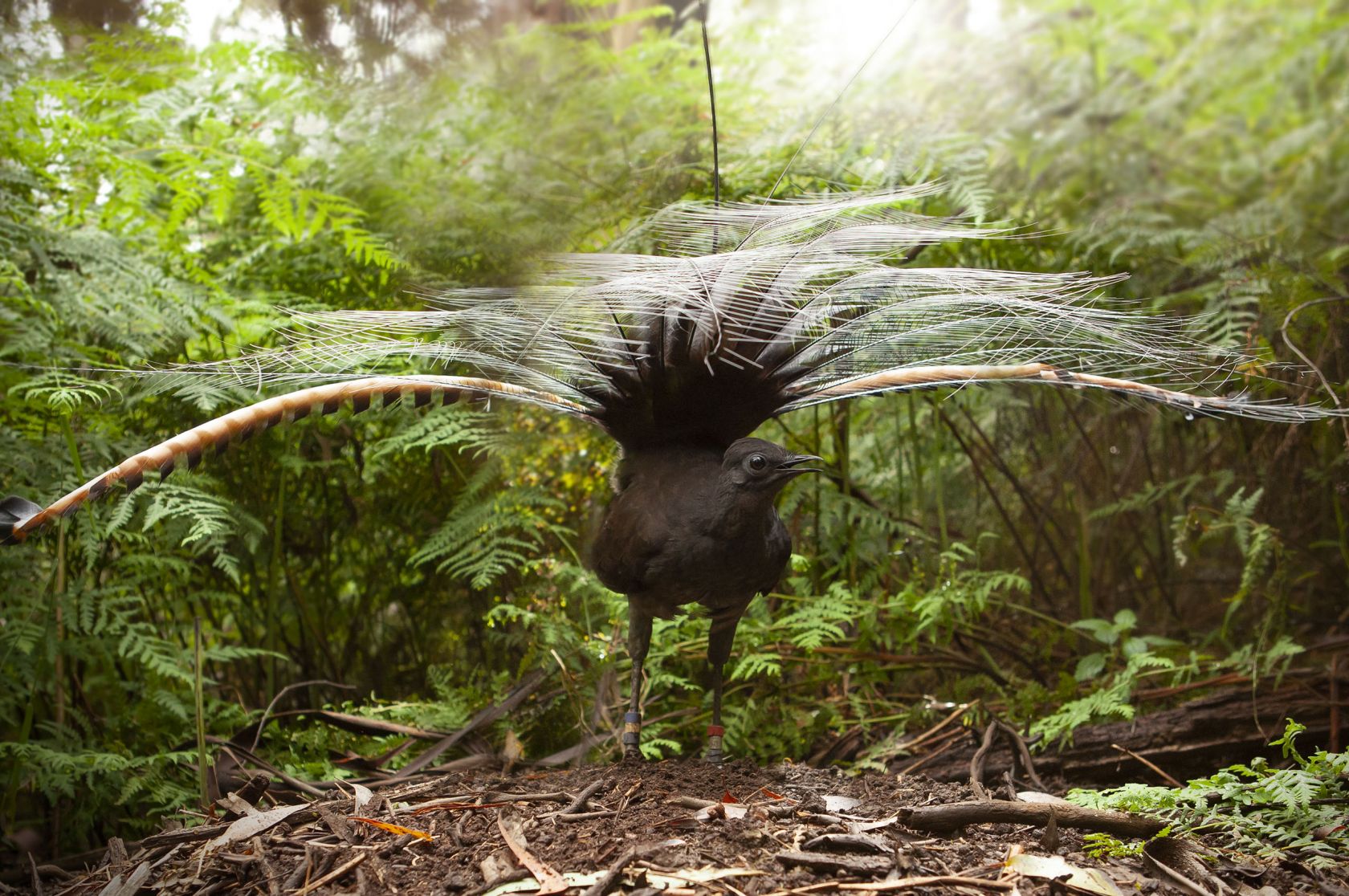The photograph captures an exotic black bird standing in a lush, forested area. The bird's body faces the camera, while its head is turned so that only its right eye, built into the side of its head, is visible. It has a fairly short beak, with the upper portion longer than the lower one. The bird's long, stick-like legs are prominently black, though they may have tags suggesting human tracking.

The bird’s impressive tail feathers, which arch out to the sides like those of a peacock, are a striking feature. While not as expansive as a peacock's, the tail feathers are predominantly light gray, with thicker, brown ridge-like patterns along the edges. These intricate feathers extend gracefully to the right and left.

Surrounded by dense vegetation consisting mainly of ferns and other green leafy shrubs, the setting has plentiful natural light filtering through, illuminating the scene. The ground is covered with sticks, brown soil, and fallen leaves, adding to the authentic forest atmosphere. The clarity and brightness of the image highlight the bird against its verdant backdrop, making each detail vividly clear.